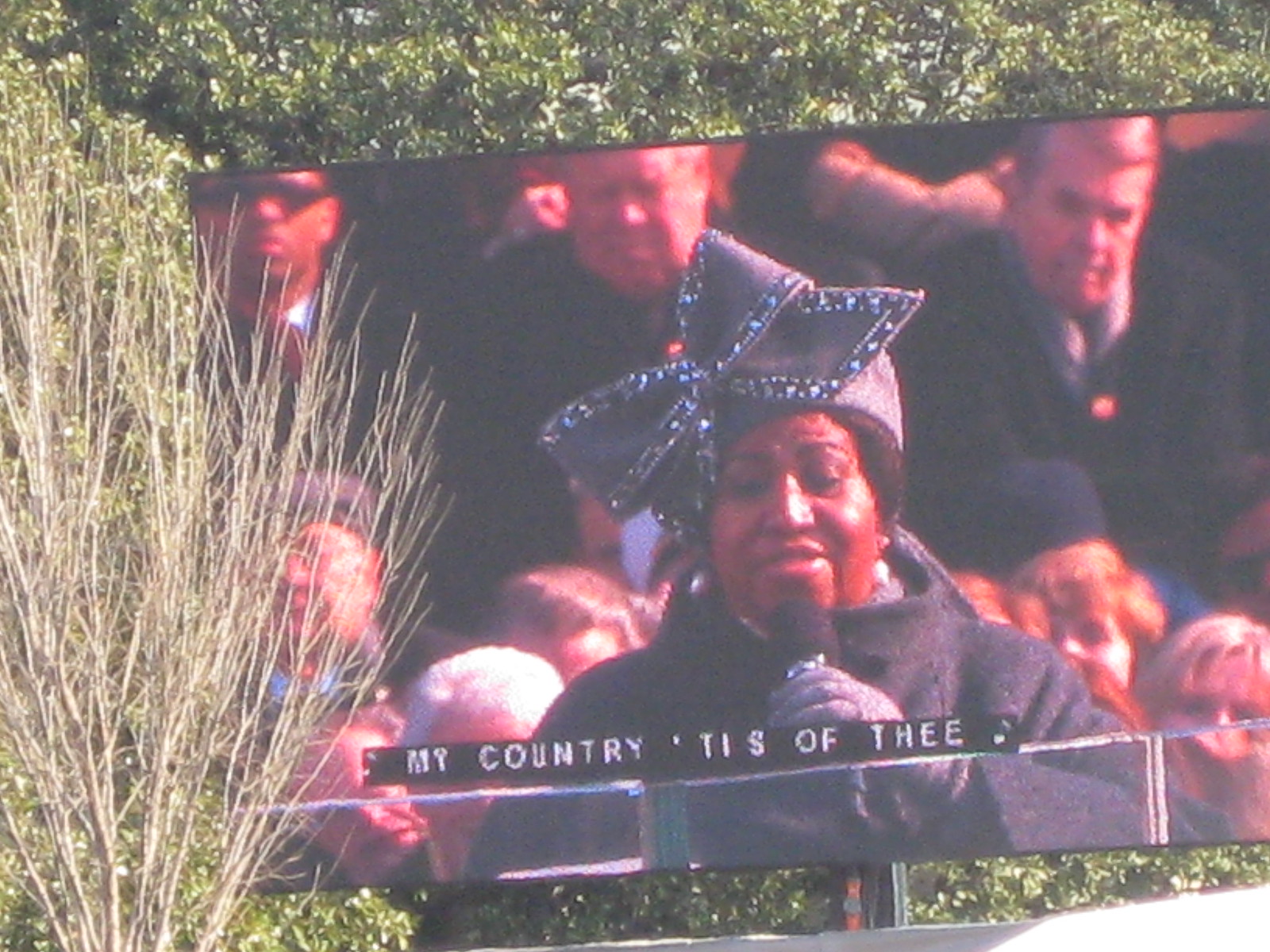In the photograph, a large outdoor screen or television set dominates the frame, set against a backdrop of leafy green trees and a leafless tree with many branches partially obscuring the screen. The focal point is the image on the screen, depicting a black woman who appears to be singing, as indicated by the closed captioning, which reads "My Country Tis of Thee" alongside musical note symbols. The woman is dressed in a large black wool coat, a hat adorned with a large black bow encrusted with diamonds, and a single visible glove. Her eyes are closed, and she holds a microphone, seemingly engrossed in her performance. In the background, various onlookers seated and partly obscured by the woman can be seen. Their formal attire, including long coats, adds to the solemn and serious atmosphere of the scene. The trees surrounding the screen enhance the outdoor setting, creating a juxtaposition between the natural environment and the technology of the large screen.